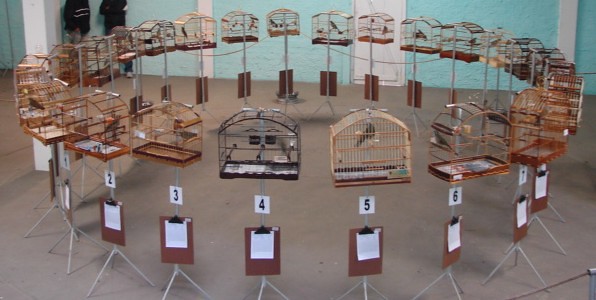The image presents an indoor setting with light turquoise-blue walls and a concrete floor. Central to the scene is a circular arrangement formed by numerous bird cages, each perched atop thin tripod stands. These cages come in various shades including black, brown, tan, and beige, with each cage housing a bird. Directly beneath every cage is a numbered white square with thick black text, ranging from at least 1 to 7, and potentially extending much higher. Each number is accompanied by a clipboard featuring a dark brown background and a white paper secured by a black clip, though the writing on the paper remains illegible due to distance. The stands, made of slender poles, uniformly support the bird cages and numbers. In addition to the cages and stands, there are two individuals visible in the corner of the image, identifiable by their black jackets but with their faces obscured from view. The backdrop is further enhanced by the presence of white pillars or a door on the turquoise wall, adding architectural detail to the setting.